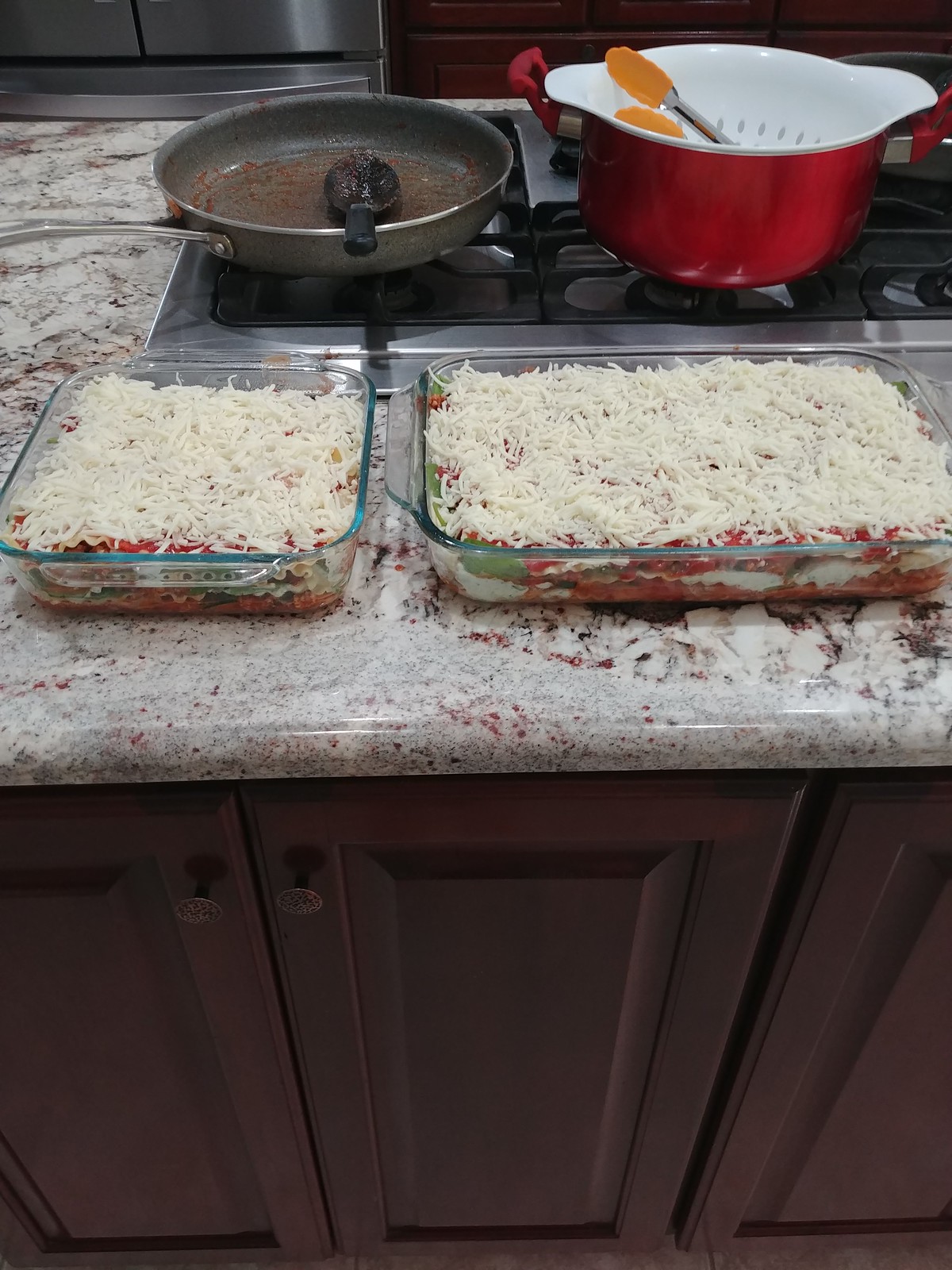The image showcases a kitchen scene centered around a prominent island counter with dark brown cupboards and a marble countertop featuring a variegated palette of tans, browns, reds, and some grays. Resting on this countertop are two clear, oblong baking dishes filled with uncooked lasagna, meticulously layered to reveal visible whites of pasta and sauce interspersed with reds of the tomato-based sauce. Both dishes are topped generously with shredded mozzarella cheese, indicating they are prepped but not yet baked, as the cheese remains unmelted. Above the countertop is the stovetop, which features metal construction with black grates. On the stove sits a red kettle with a strainer inside and a pair of orange-handled metal tongs. Beside it is a metal frying pan containing a black plastic spoon and some remnants of food. This detailed setup, with everything in place, suggests a moment captured just before the lasagna dishes are to be baked, highlighting the preparatory stages of a delicious meal in a well-organized kitchen setting.